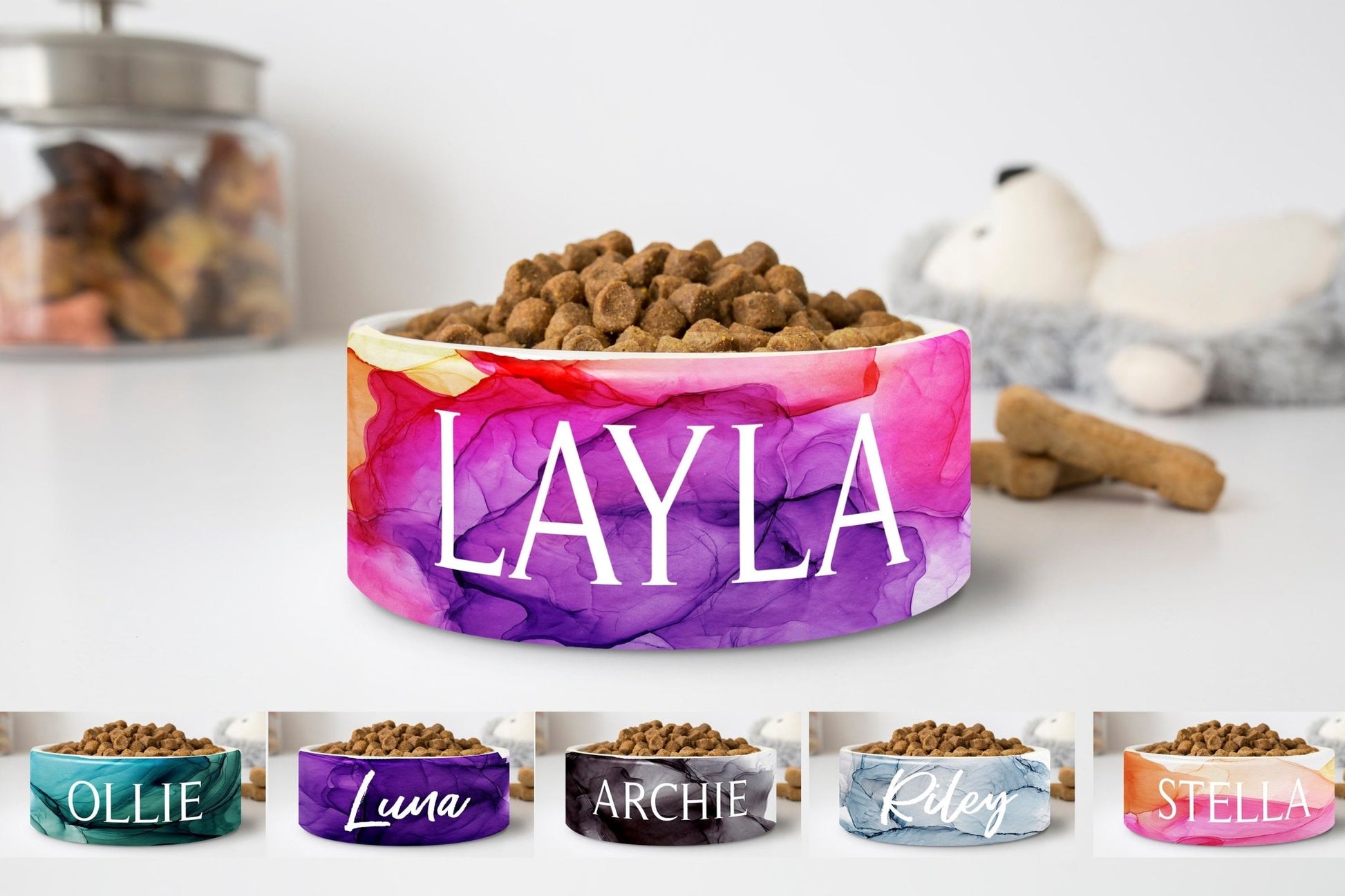Poster Advertisement for Personalized Pet Food Bowls

At the center of this vibrant poster, a large pet food bowl takes precedence, proudly showcasing the name "Layla" in striking white lettering. The bowl is brimming with kibble, set against a rich, colorful backdrop blending hues of pink, red, purple, and white. To the right of Layla's bowl, two crossbones add a playful touch.

In the background, slightly out of focus, a plush stuffed animal adds a cozy ambiance, while to the left, a vacuum container holds an unidentifiable object, contributing to the homey setting.

At the bottom of the poster, five additional customized bowls are displayed, each filled with kibble and featuring different names—Ollie, Luna, Archie, Rylee, and Stella. These bowls are presented with various backgrounds and color schemes, highlighting the personalization options available for your pet's feeding essentials.